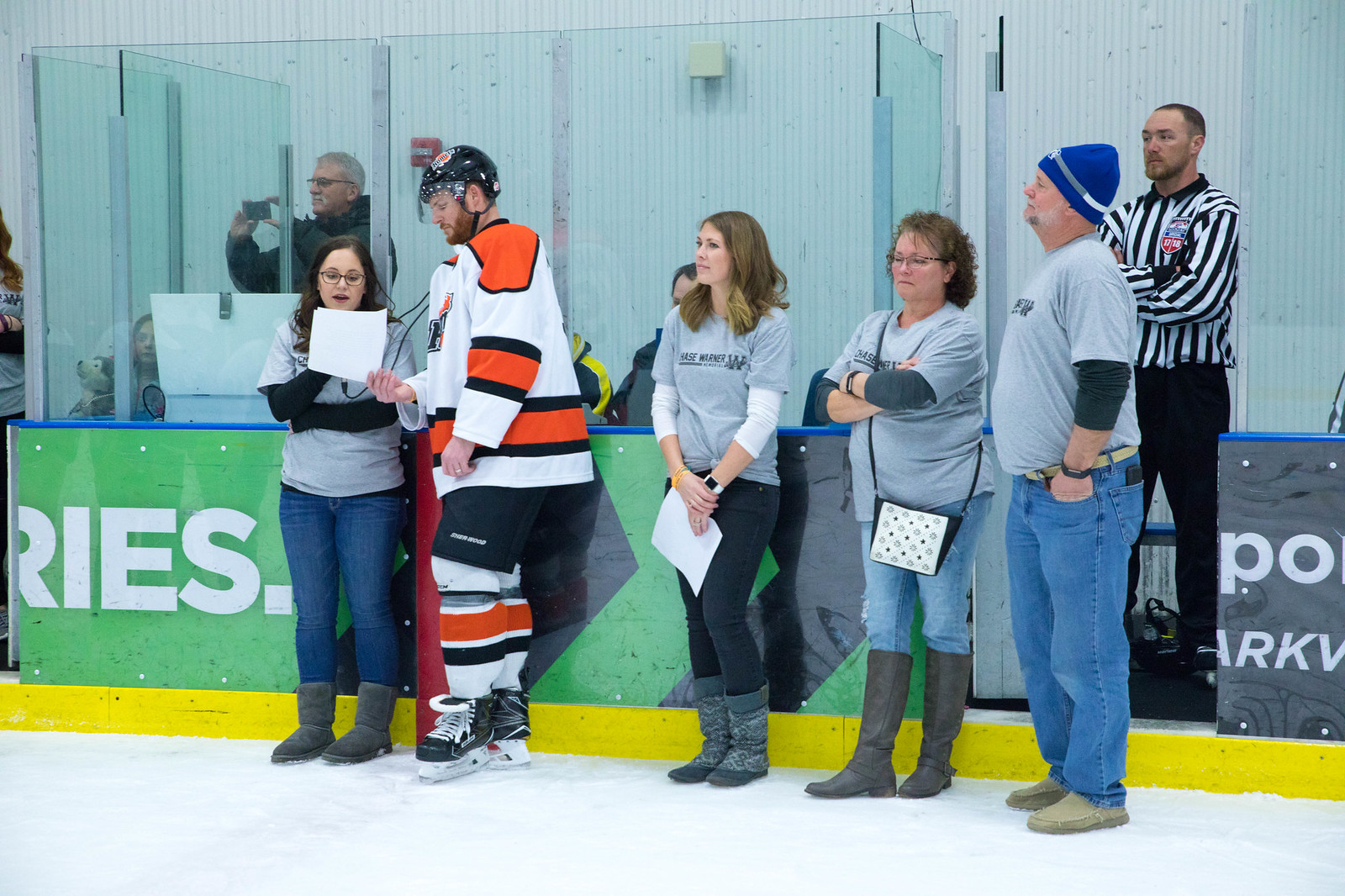In this image taken at an indoor ice hockey stadium, several people stand on the ice near a glass barrier. Prominently in the center is a hockey player, dressed in a white uniform with orange and black stripes, and wearing a black helmet. He is a white man with a brown beard and is holding a piece of paper. To his left stands a woman with glasses, wearing a gray t-shirt with black undersleeves, blue jeans, and gray boots. She appears to be speaking into a microphone, looking at the paper the hockey player is holding. 

On the right side of the image, two more women are visible. One, with shoulder-length brown hair, is wearing a gray t-shirt over a white long-sleeve shirt, black pants, and gray boots. She holds a sheet of paper and is wearing a smartwatch. Next to her, a woman with short hair and glasses is dressed in blue jeans, gray knee-length boots, and a gray t-shirt over a dark gray long-sleeve shirt, along with a small purse slung over her shoulder.

Also on the right, an older man wearing a blue cap, gray t-shirt over a black long-sleeve shirt, blue jeans, and light green shoes, stands observing. He is joined by another man in the background, identifiable as a referee wearing the traditional black and white striped uniform and black pants. Behind them is a cabin with a large desktop screen, possibly for scorekeeping, and inside it, another gentleman taking photos with his camera. A green and yellow banner with partially visible letters hangs outside the cabin. The scene is animated with the buzz typical of a live hockey event.